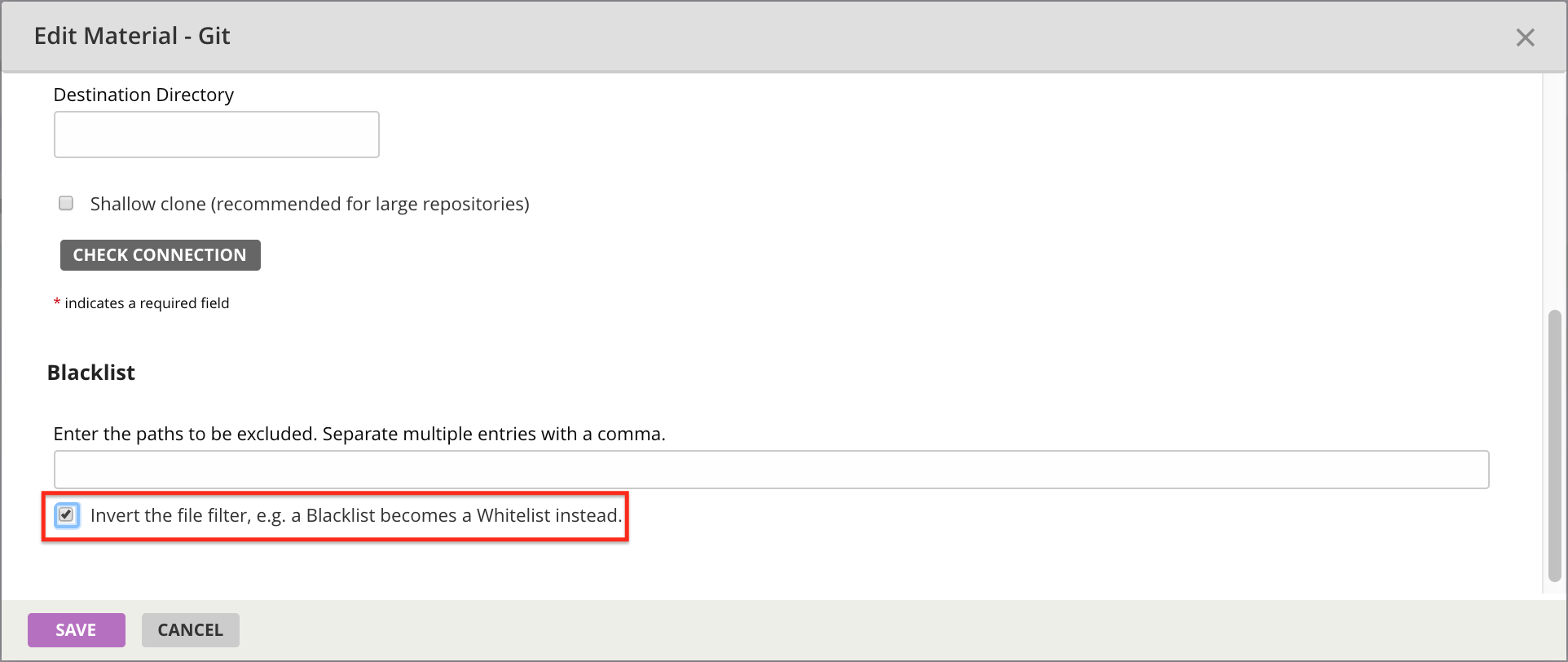This image displays a section of a Git management application interface, specifically focusing on the edit options for material configurations. 

At the top, the title **"Edit Material - Git"** is displayed in a grayed-out font, indicating the current section being edited. Below it, there is an empty text box labeled **"Destination Directory"** where users can input a path but, in this case, remains unfilled. 

Adjacent to this, there's an unchecked checkbox labeled **"Shallow clone (recommended for larger repositories)"**. Next to that is a **"Check Connection"** button, styled in a grayish-black.

A small, red asterisk icon is present, signifying that the field is required. Moving further down, there is bold text labeled **"Blacklist"**. Beneath this label, an instruction reads **"Enter the paths to be excluded, separate multiple entries with a comma,"** followed by an input box meant for user entries.

Below this input box, a checkbox is highlighted by a red rectangular outline and is checked. The label reads **"Invert the file filter, e.g., a blacklist becomes a whitelist instead."** This checkbox is surrounded by a faint blue square.

Finally, at the bottom of the interface, there is a **"Save"** button in purple and a **"Cancel"** button in gray. The majority of the interface is set against a plain white background, giving it a clean and simple appearance.

Overall, this interface appears to be part of a Git management application, possibly GitHub, focused on setting up various connection parameters, although no specific data or paths have been entered in this particular instance.